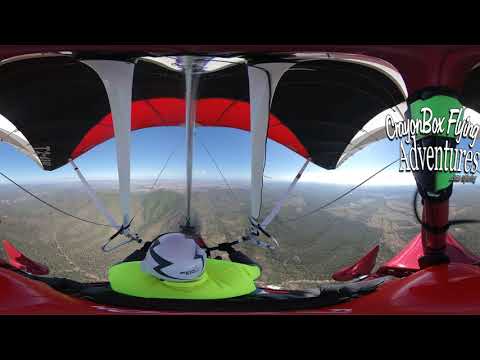The photograph captures a high-altitude adventure scene featuring a person parachuting, framed by a vivid panoramic view of a mountainous landscape. The image is taken from above, offering a unique perspective. The parachute is predominantly red with black and white details, enveloping the individual. They are equipped with a white helmet adorned with blue lightning bolts, black gloves, and a neon yellow safety vest. The person's position in the air provides a sweeping view of the grey-brown mountains below and a slice of bright blue sky above, dotted with white clouds and sunlight. On the right side of the image, the words "Crayon Box Flying Adventures" are inscribed in white text, with "Adventures" styled in a serif font beneath "Crayon Box," which appears in a more casual, handwritten script.